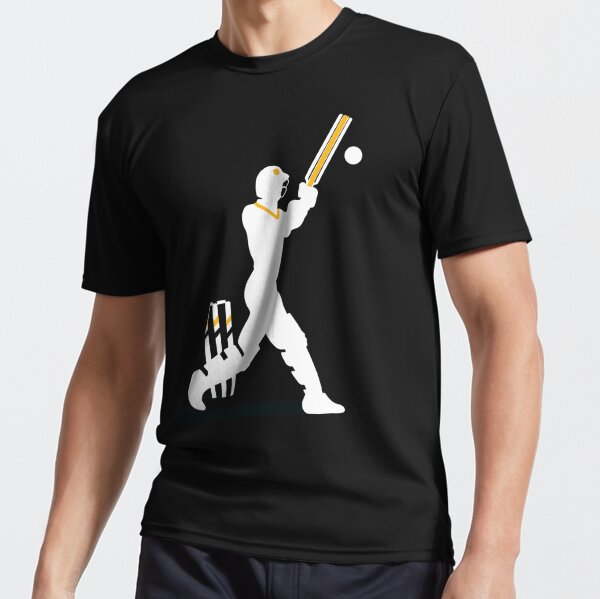This image is designed for a website selling t-shirts. It features a Caucasian male model, shown from the neck down, wearing a black t-shirt that prominently displays a sports-related design. The focus is on the t-shirt, which features a detailed, white silhouette of a cricket player in mid-swing with a yellow cricket bat. The player's profile is rendered in white, with additional details such as leg pads and shoes, as well as three cricket stumps behind him, accentuating the cricket theme. The yellow accents are also present on the helmet and around the neck of the player, providing a vivid contrast to the black t-shirt. The arms and part of the pants of the model are also visible, enhancing the overall view of the t-shirt, which is posed to highlight its design for potential buyers.